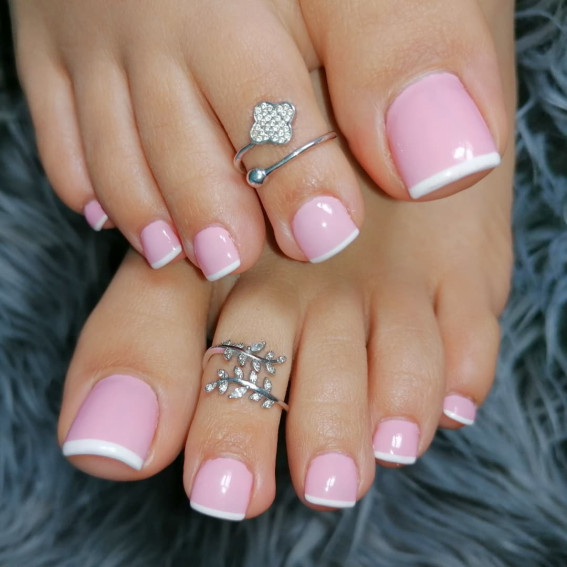The image depicts a pair of freshly manicured feet, resting on a soft, satin-like aqua or teal-colored sheet. Each toenail features a French manicure with a light pink base and crisp white tips, meticulously cut square on the edges. Both feet possess toe rings on the index toes, one designed as a vine leaf with rhinestone accents, and the other adorned with a ball and clover motif embedded with rhinestones. One foot is elegantly crossed over the other, showcasing the exquisite manicure and decorative toe rings. The toes are notably elongated and finger-like, giving the feet a unique, hand-like appearance.